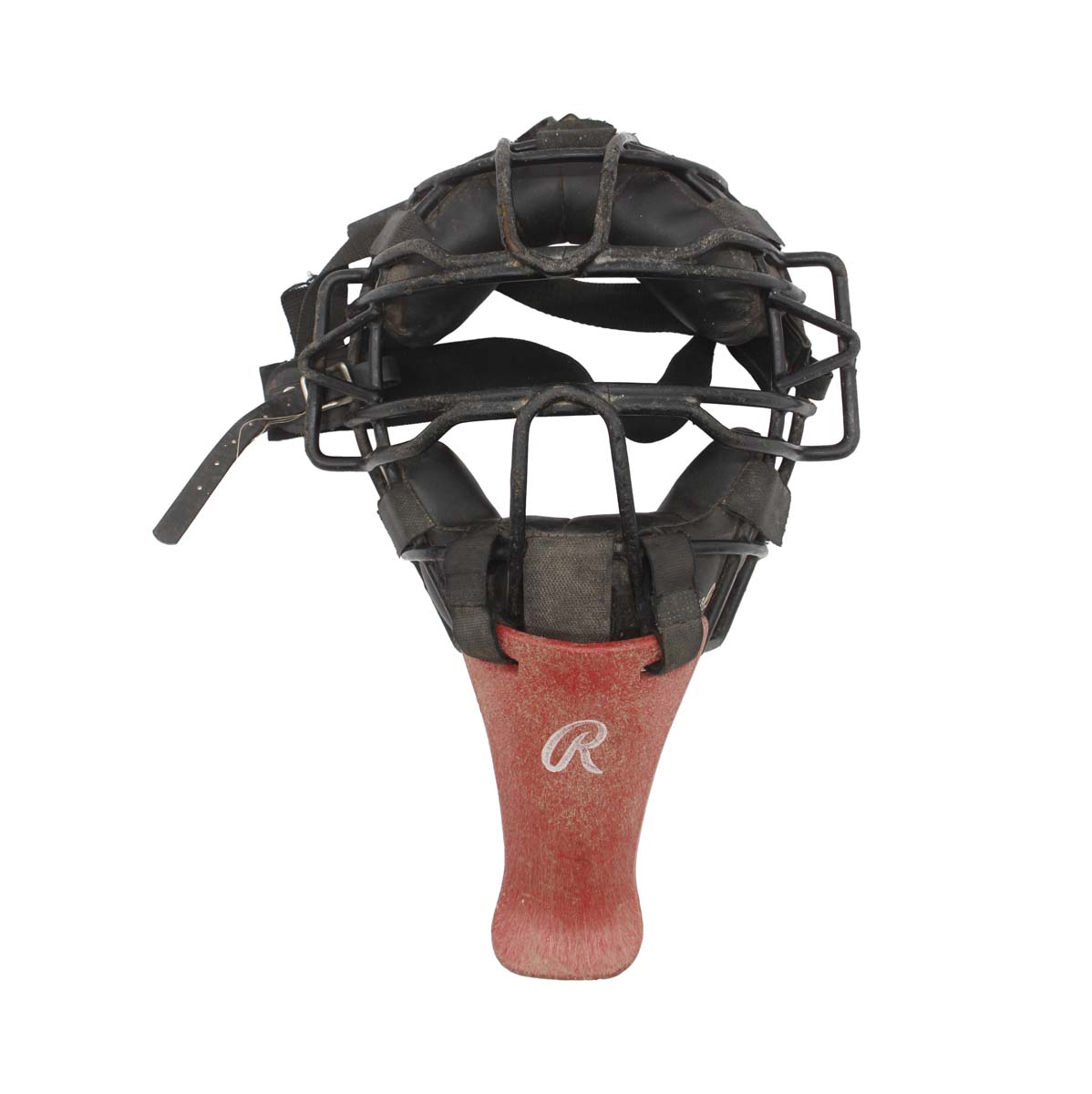This image captures an old, well-used black catcher's mask, positioned centrally against a white background. The mask features thick black padding at the top and bottom, with black straps on the left side for fitting. A metal cage frames the eye area, forming a rectangular structure, with additional metal loops at the top and bottom for secure fastening. Notably, the mask includes a red plastic throat guard dangling from the bottom, emblazoned with a white, cursive 'R' logo, likely representing the Rawlings brand. The red throat guard exhibits a whitish-brown wear and tear, indicating extensive use. The black metal cage also shows various scuff marks, reinforcing the mask's heavy use and age.